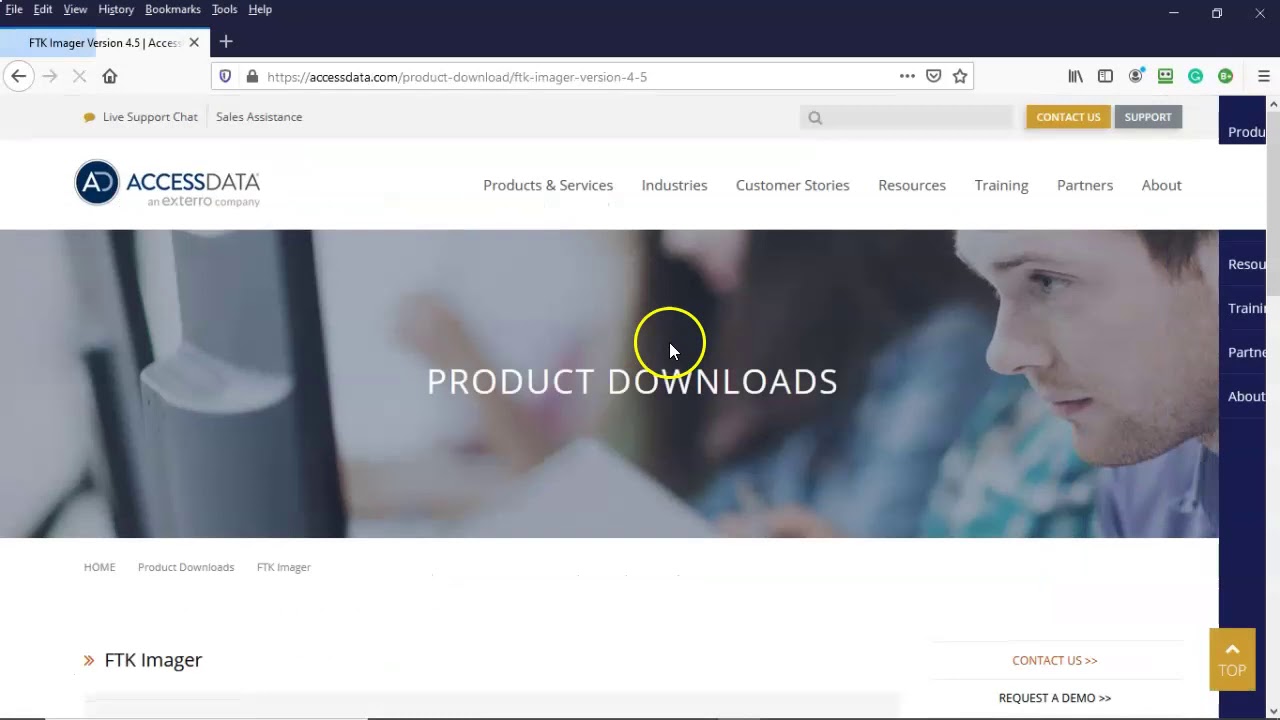A screenshot of a web browser with a dark theme—likely black or dark navy blue—displays a single tab titled "FTK Manager Version 4.5," accompanied by the URL: "https://dataaccess.com/product-download/FTK-manager-version-4-5." The mid-section of the page features navigation elements, including a live support chat and sales assistant options on the left and a search bar on the right. Adjacent to these, there are a mustard yellow "Contact Us" button and a grey "Support" button.

Below this navigation area, a photograph captures a close-up of a man, revealing his head and shoulders as he looks at a computer screen. In the background, the blurred image of another individual can be discerned, focus drawn away by a yellow circular cursor. Further down, the webpage's main content is organized by breadcrumbs reading "Home > Product Downloads > FTK Manager" on a white strip. Beneath, the labels "FTK Manager," "Contact Us," and "Request a Demo" are prominently displayed.